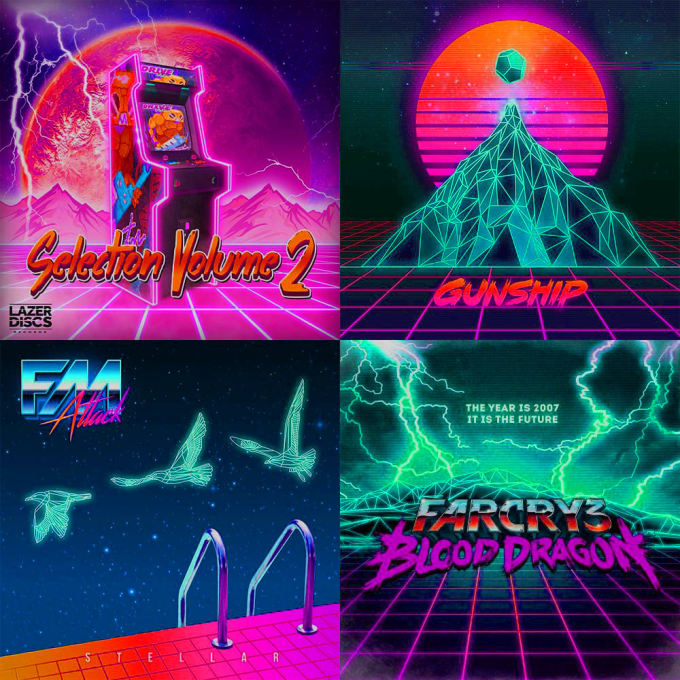This vibrant, digitally illustrated square image is divided into four distinct yet stylistically cohesive square sections, all boasting an '80s-inspired neon color palette of magenta, purple, dark blue, and green. 

In the upper left quadrant, an old-fashioned pinball machine is set against a stormy sky with lightning bolts, accompanied by the text "Selection, Volume 2" in red font. The bottom corner of this segment also features the phrase "Laser Discs."

The top right section showcases a geometrically stylized mountain with a sphere, reminiscent of a sun, casting its glow from behind. This segment bears the caption "Gunship" in striking red letters.

The bottom left quadrant depicts a poolside scene complete with a pool ladder and a trio of geometrical birds soaring through a starlit dark blue sky. The words "FM Attack" are prominently displayed in the upper left corner.

The final section, located in the bottom right, features an electrifying sky filled with lightning over a black floor segmented with pink. The text declares, "The year is 2007, it is the future," followed by the title "Far Cry 3 Blood Dragon" in bold white font, laid over a magenta grid pattern.

Together, these segments create a vivid, retro-futuristic collage that appears to reference various video games and themes.